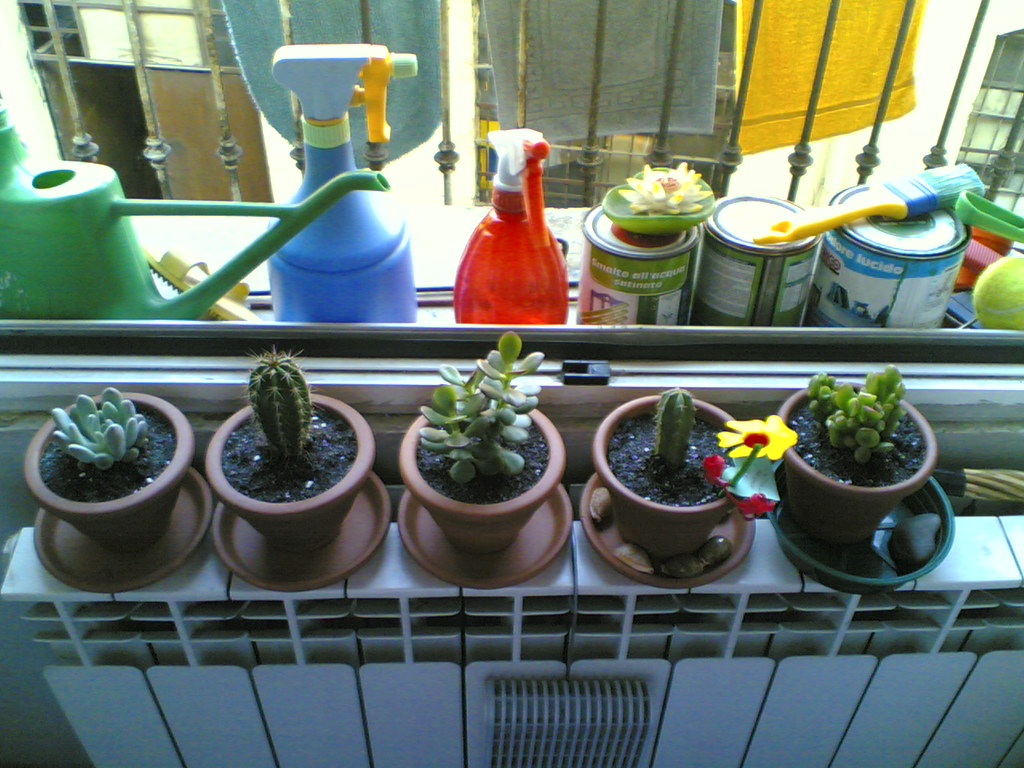This photograph captures an indoor setting featuring a neatly arranged row of six cactus plants on brown pots placed on a white radiator ledge in front of a window. Each pot is dark with soil, resting on saucers. The cacti vary in type, from a small light green cactus with multiple lumps on the far left, to a tall cylindrical one with brown spikes, another with numerous green leaves or spines, a small circular cactus, and a complex one with green nubs on the far right. One of the cacti has a small fake red and yellow flower inserted into it, along with some stones scattered in its dish. 

In the background, through the window, a variety of objects can be seen. Spray bottles in blue and red with nozzles, a green watering can, and a few cans of paint or stain with a resting paintbrush are visible on the windowsill. Additionally, a small fake lily pad with a flower and some fabrics – a blue rug, a gray rug, and a yellow towel – are draped over a decorative railing. The scene is framed by hints of an urban environment outside, with distant buildings and windows indicating a vantage from a city apartment.